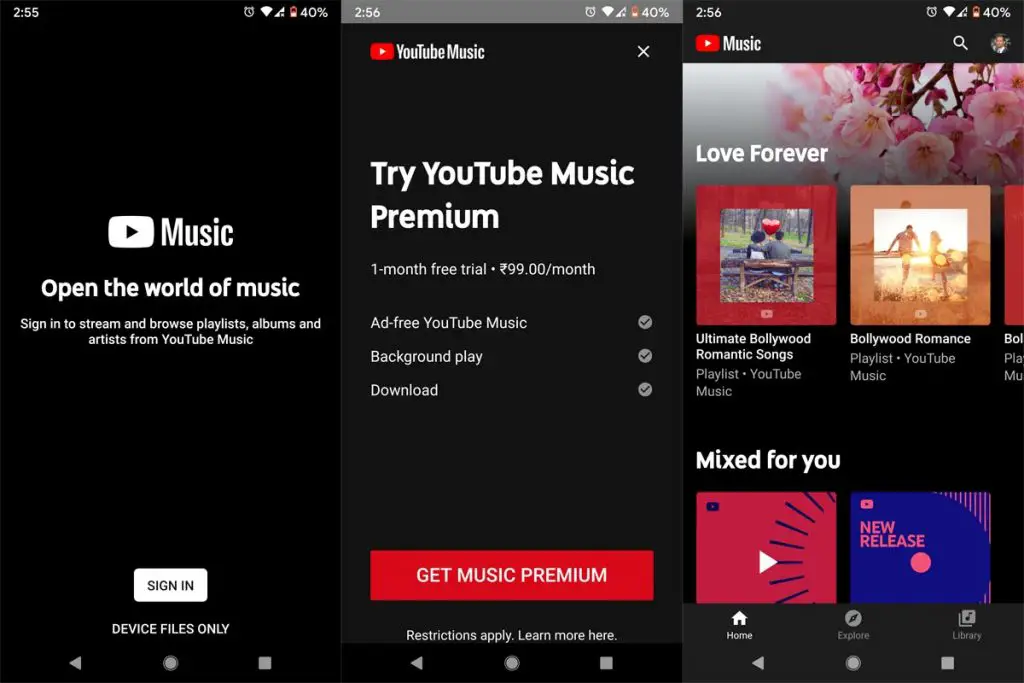The image is a composite of three screenshots from a cell phone, arranged side by side against a predominantly black background. The timestamps at the top indicate that the left screenshot was captured at 2:55, while the middle and right screenshots were taken at 2:56.

In the first screenshot on the left, white text superimposed on the dark background reads: "Open the world of music. Sign in to stream and browse playlists, albums, and artists from YouTube Music." Below this text, a white play button with a black triangle and a "Sign In" button are prominent, alongside a note stating "Device files only."

The middle screenshot promotes a trial offer, displaying the message: "Try YouTube Music Premium, one month free trial, $9.99 a month." It highlights features such as "Ad-free YouTube Music," "Background play," and "Download," each accompanied by a gray check mark.

The third screenshot on the right features text that reads "Love forever" and "Mixed for you," with several small squares indicating music playlists or albums.

Overall, the composite image appears to be promoting the YouTube Music service, showcasing various features and benefits to entice users to sign up and explore its offerings.